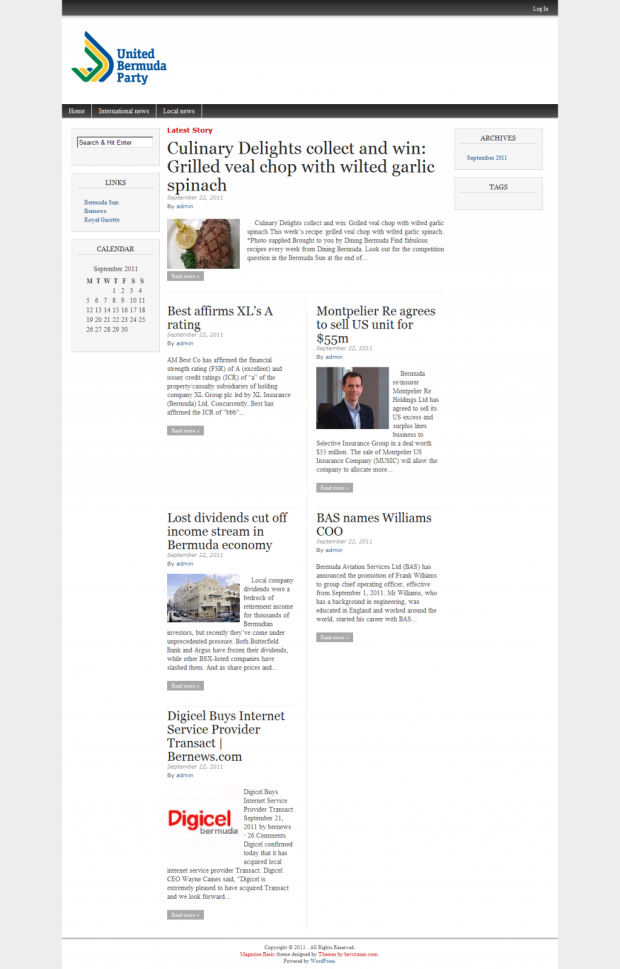The image is a vertically rectangular frame bordered on the left and right sides by gray. Inside the border, the main image depicts a webpage from the "United Bermuda Party" website. The image captures an elongated, scrolling screenshot of the webpage, making the text appear small, yet some headlines are still legible. These headlines include "Culinary Delights Collect and Win," "Grilled Veal Chop with Wilted Garlic Spinach," "Best Affirms Excel's A Rating," "Montpelier Ray Agrees to Sell U.S. Unit for $55M," "Lost Dividends Cut Off Income Stream in Bermuda Economy," "BAS Names Williams COO," "Digicel Buys Internet Service Provider Transact," and "BurnNews.com." Within the webpage, there are multiple images corresponding to some of these stories: a visual accompanying the "Culinary Delights Collect and Win" article, another image related to "Montpelier Ray Agrees to Sell U.S. Unit for $55M," and one more paired with the "Lost Dividends Cut Off Income Stream in Bermuda Economy" news.